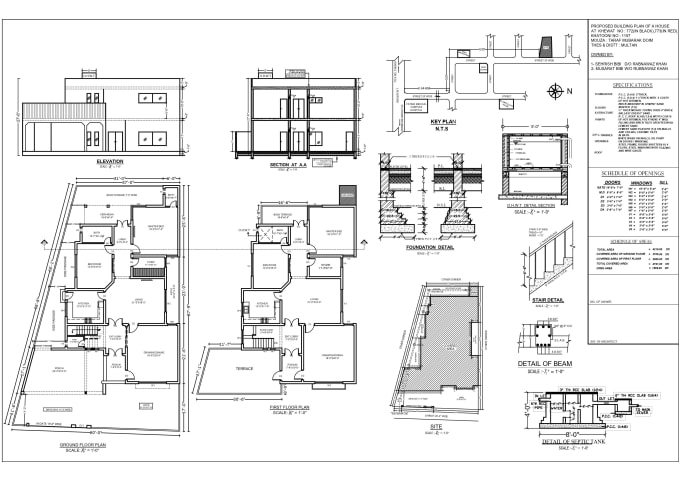The image is an intricately detailed architectural drawing of a house, showcasing both exterior and interior views. Dominating the layout are multiple schematic drawings that include around ten different perspectives of the house, such as elevated and back views, as well as top-down floor plans. Notable detailed sections highlight elements like a staircase, a cross-section of a beam, and a septic tank located at the bottom right corner. The drawings are predominantly black on a white background, featuring straight-lined and precise architectural markings. While the drawing includes a legend and various labels for each view, which run down about two-thirds of the right-hand side and into a long rectangular box, the text is largely unreadable due to its small size. Despite this, the diagram comprehensively conveys the structural and spatial arrangement of the house, distinguishing doorways, windows, and various rooms within the building.